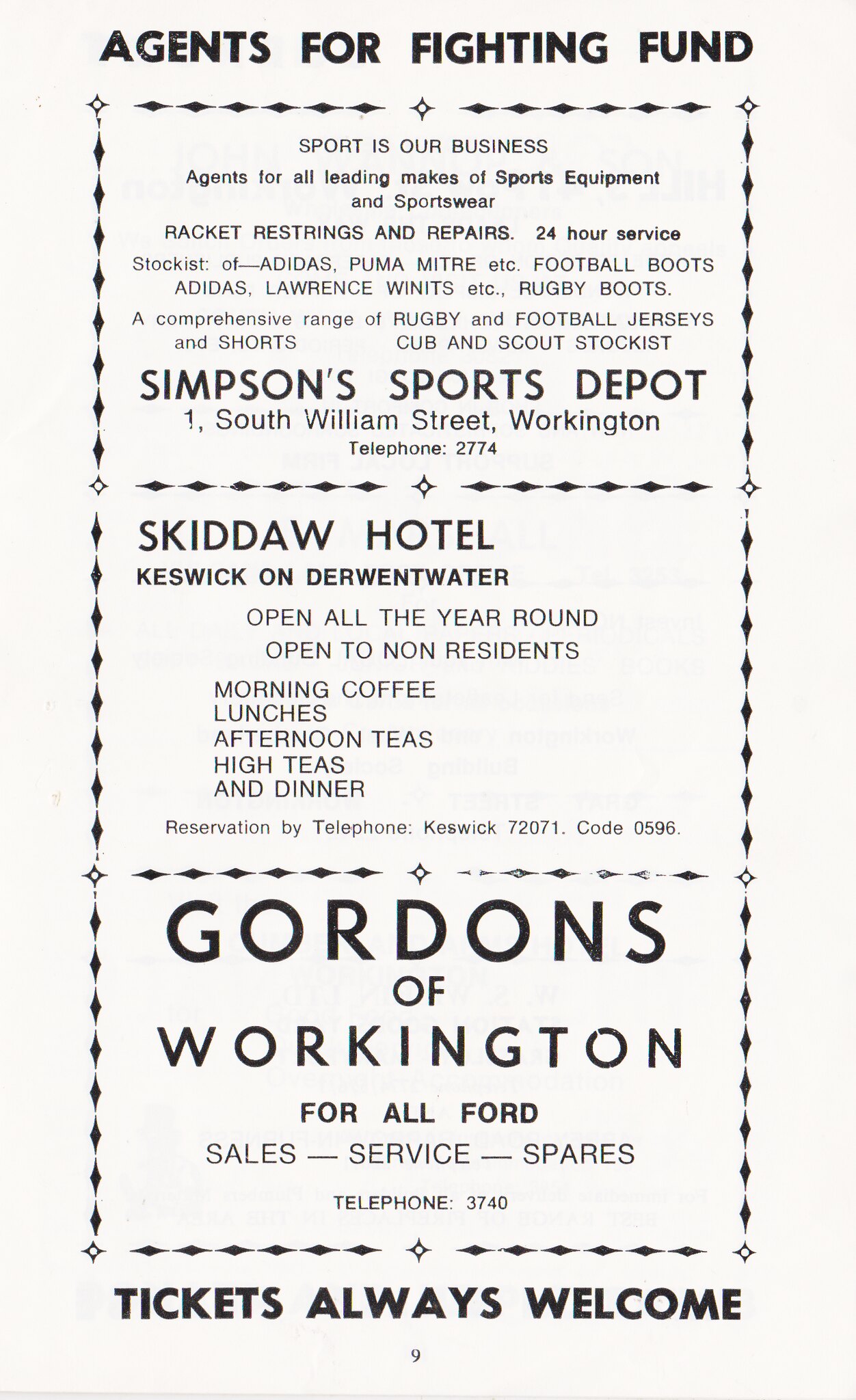This black and white advertisement, titled "Agents for a Fighting Fund," consists of three distinct sections set against a white background. At the top, in bold black text, the title is prominently displayed. The first section features an ad for Simpson's Sport Depot including its slogan, "Sport is our business," along with the address and contact number located at South William Street, Workington. The second section advertises the Skadaw Hotel, situated in Keswick on Derwent Water. It notes the hotel is open year-round, welcomes non-residents, and offers morning coffee, lunches, afternoon teas, high teas, and dinners, with reservations available via telephone at Keswick 7271 (code 0596). The third section promotes Gordon's of Workington, detailing services such as sales, service, and spares for Ford vehicles, with the contact number 3740. At the very bottom of the image, "Tickets always welcome" is emphasized in black text, adding a welcoming touch to the advertisement.